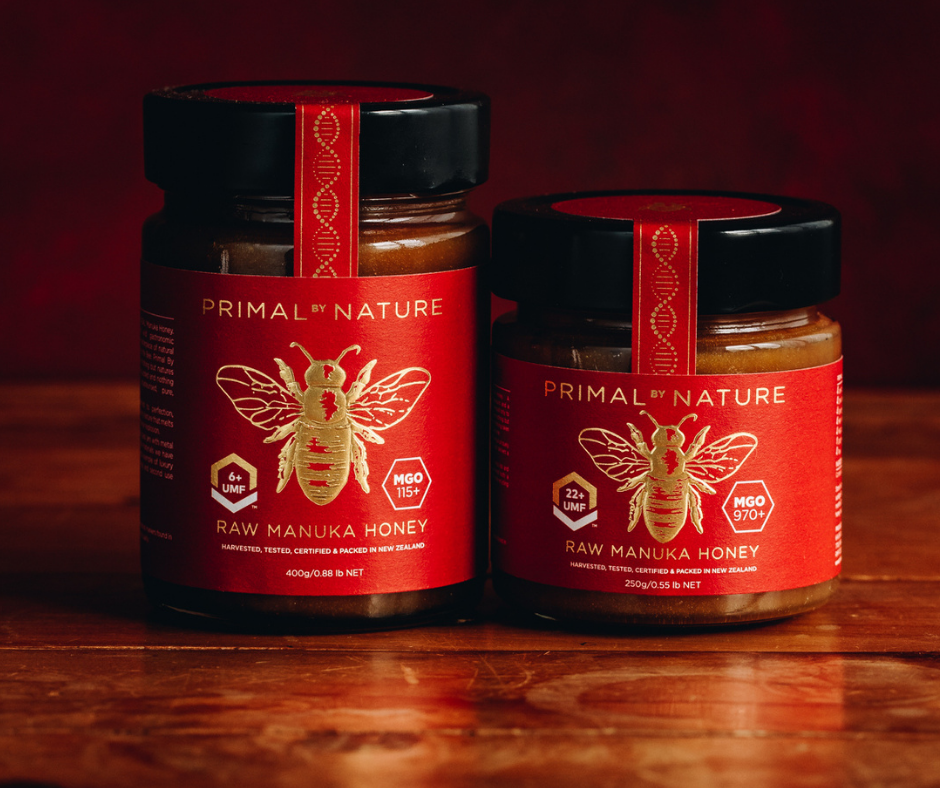This detailed image features two jars of raw Manuka honey, prominently displayed on a shiny, dark wooden surface that appears to be either a table or a countertop. Both jars have black lids and striking red labels with gold detailing. The jar on the left is slightly taller, labeled as containing 400 grams (0.88 pounds) of honey, while the jar on the right holds 250 grams (0.55 pounds). The labels, belonging to the brand "Primal by Nature," feature a gold-foil butterfly illustration with its wings spread, accompanied by details about the honey: harvested, tested, certified, and packed in New Zealand. A narrow red strip, embellished with a gold double helix, runs up from each main label and over the lid, serving as a safety seal. The background is somewhat blurry, revealing hints of dark brown and black tones in the wood, complementing the reddish-brown color palette of the foreground.